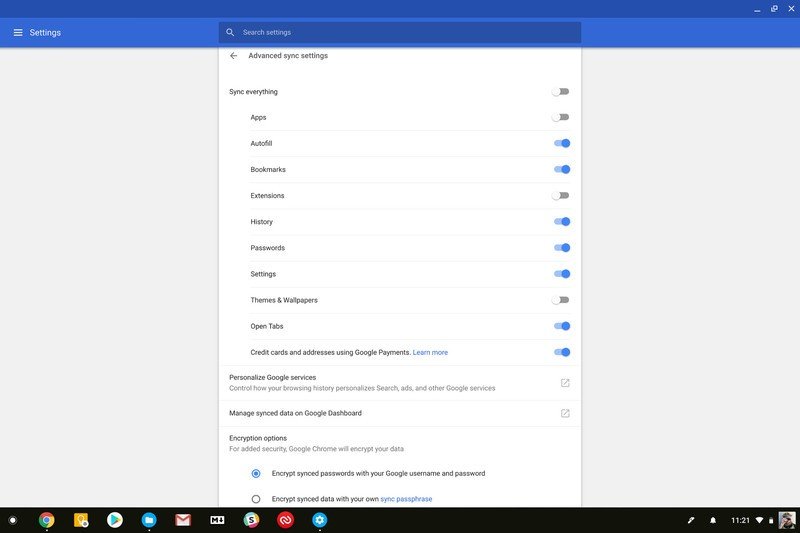The top section of the image features a dark blue background. Directly below this dark blue area is a lighter blue section with the word "Settings" displayed on the left side. Situated towards the top, there is a dark blue search box containing the text "Search settings."

Below the search box, the background transitions to gray, containing a prominent white box. This white box lists various terms aligned on the left side, each accompanied by a toggle switch on the right. Some of these toggles are switched on, while others are off.

The terms listed include:
- Advanced sync settings
- Sync everything
- Apps
- Autofill
- Bookmarks
- Extension
- History
- Passwords
- Settings
- Themes and wallpaper
- Open tabs
- Credit cards and addresses using Google Payments
- Personalize Google services

Additionally, the white box contains the following text elements:
- "Learn more"
- "Control how your browsing history personalizes search ads and other Google services"
- "Manage sync data on Google dashboard"
- "Encryption option for added security: Google Chrome will encrypt your data, encrypt sync password with your Google username and password."